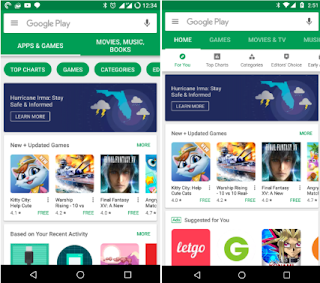This image depicts two screenshots of a cellphone screen, showcasing the Google Play Store interface. Both screenshots have a predominantly green header at the top, indicating the Google Play search area. On the left, the time displayed is 12:34 PM, whereas on the right it is 2:51 PM, with noticeable differences in the battery and other status icons, suggesting they might be from different phones or instances.

The larger screenshot on the left shows that the user has navigated to the "Apps & Games" section. Below this, there's a highlighted area mentioning Florida and weather-related information. Towards the bottom of the larger screenshot, there's a list of new and updated games, including titles such as "Kitty", "Offy", "Worship", and "Fried Fantasy." The fourth game's title is partially obscured and cut off.

The smaller screenshot on the right mirrors much of the same content but with less clarity and a slightly smaller green header. The layout and app icons appear consistent with the left screenshot, albeit resized. Overall, this comparison provides a detailed glimpse into the user’s Google Play Store interface at two different times.